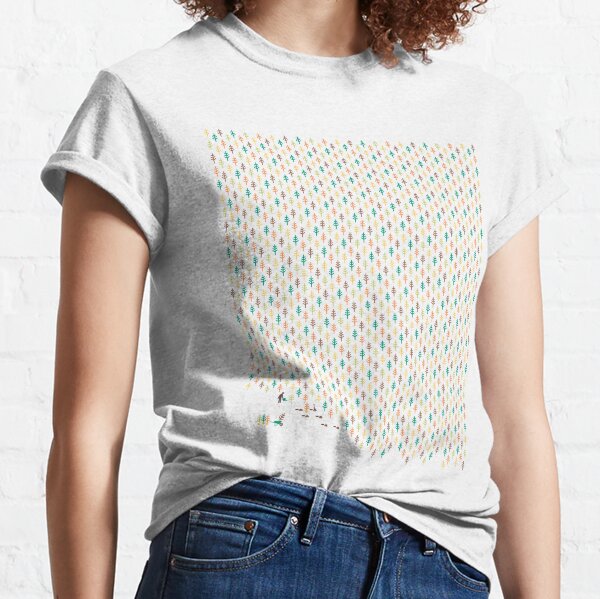The image features a young light Caucasian woman with shoulder-length, very curly, reddish auburn hair. She is modeling a white t-shirt with short sleeves that extend to her biceps. The t-shirt showcases a colorful checkered pattern consisting of blue, white, yellow, teal, possibly a hint of pink, and tiny trees in green, orange, maroon, and red hues, organized in a square on the front. A small indistinct figure appears in the bottom left corner of the pattern, resembling a stick man. The shirt is partially tucked into her dark blue jeans at the front and left side. Her arms dangle naturally by her sides. The background is a neutral, light gray or white wall, lending a simple and clean backdrop to the image. The photo captures her from just below her chin to slightly below her belt line, highlighting her attire and suggesting it might be for a clothing ad, perhaps from a magazine like JCPenney's.